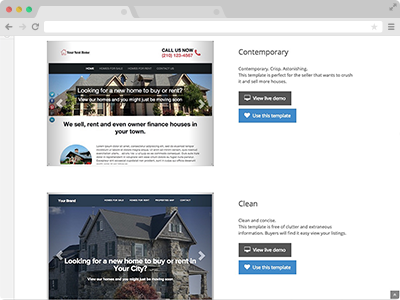A color screenshot of an unidentified webpage displays an empty address bar at the top. Prominently featured on the left side is a photograph of a home with accompanying text that reads, "Looking for a new home to buy or rent? View our homes and you might just be moving soon. We sell, rent, and even offer owner financing for houses in your town." The text below this image is too blurry to be deciphered.

At the top of the page, a section invites visitors to "Call us now," although the phone number provided is also blurred and illegible. Beside this, the word "Contemporary" is visible, followed by some additional blurry text. Among the discernible words are, "Contemporary, astonishing. This template is perfect for the seller that wants…" but the rest is unreadable. Options for "View the demo" and "Use this template" are presented.

Near the bottom of the page, another photograph of a home with gray stone walls and a gray roof is displayed, accompanied by text that states, "Looking for a new home to buy or rent in your city." Again, the text beneath is too blurry to read. To the right of this section, the words "Clean, clean and concise. This template is free of clutter and extraneous information. Sellers will find it…" appear, although the last word is too blurry to distinguish. Additionally, options for "View your listings," "View live demo," and "Use this template" are noted.